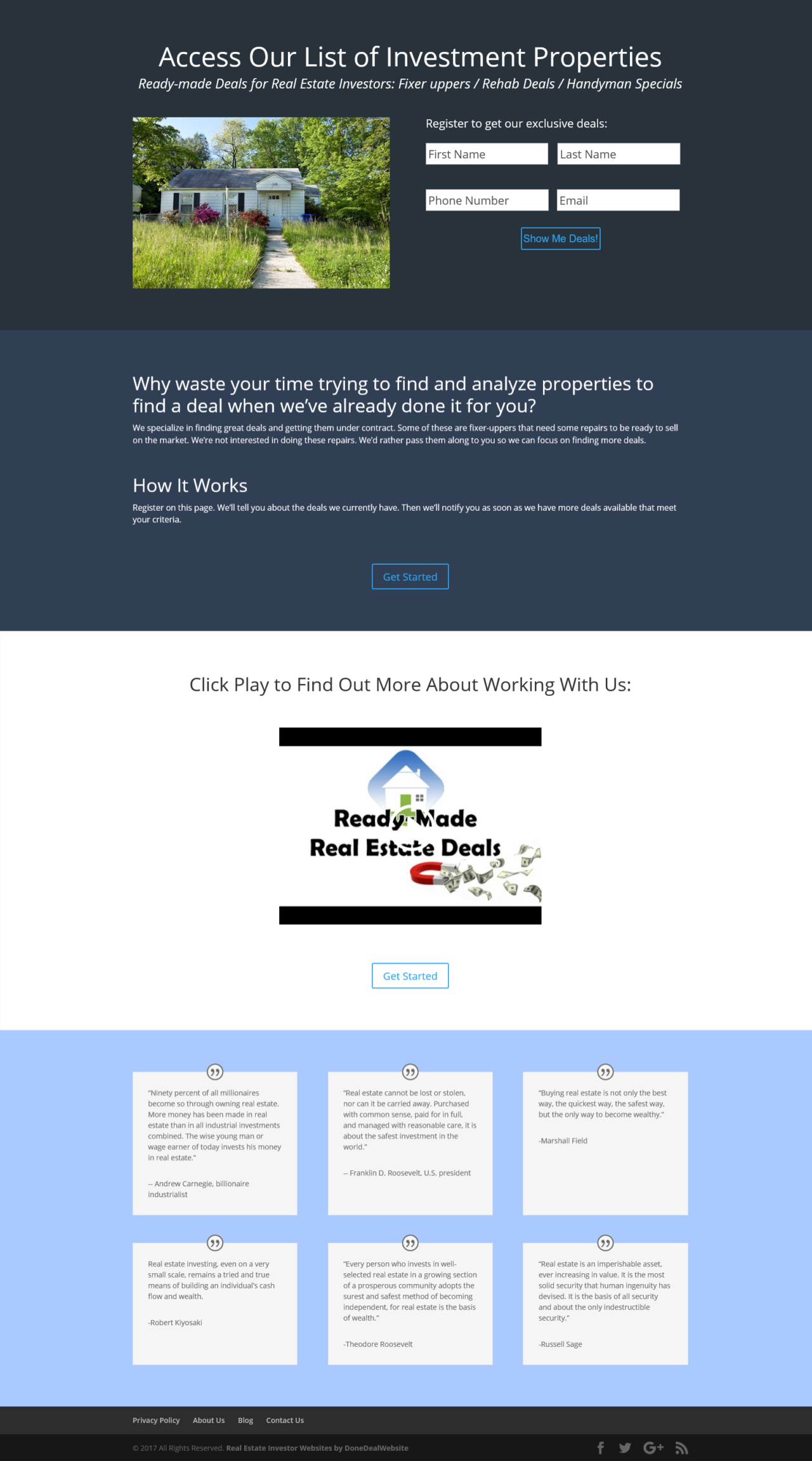The image depicts a webpage with two main sections designed for a real estate investment platform. The layout includes three distinct visuals. 

At the top section, there is a dark blue background with white text that reads: "Access our list of investment properties." Below this heading, additional text is present but is unreadable. There is a registration form with fields labeled "First Name," "Last Name," "Phone Number," and "Email," intended for users to submit their information in order to gain access to the list of investment properties. In the middle of this section, there's a small image of a somewhat dilapidated house.

The middle section has a light blue background and features motivating white text stating: "Why waste your time trying to find and analyze properties to find a deal when we've already done it for you." Following this statement, there are a few more sentences, including a subtitle "How it works," with an explanatory sentence beneath it. This area likely includes a submit button for further engagement.

Towards the bottom of the section, the text instructs "Click play for more about working with us. Read made real estate deals," accompanied by a play button, presumably for a video explaining their services. 

The final section consists of a light blue background containing six white boxes with black text, though the text is too small to be legible.